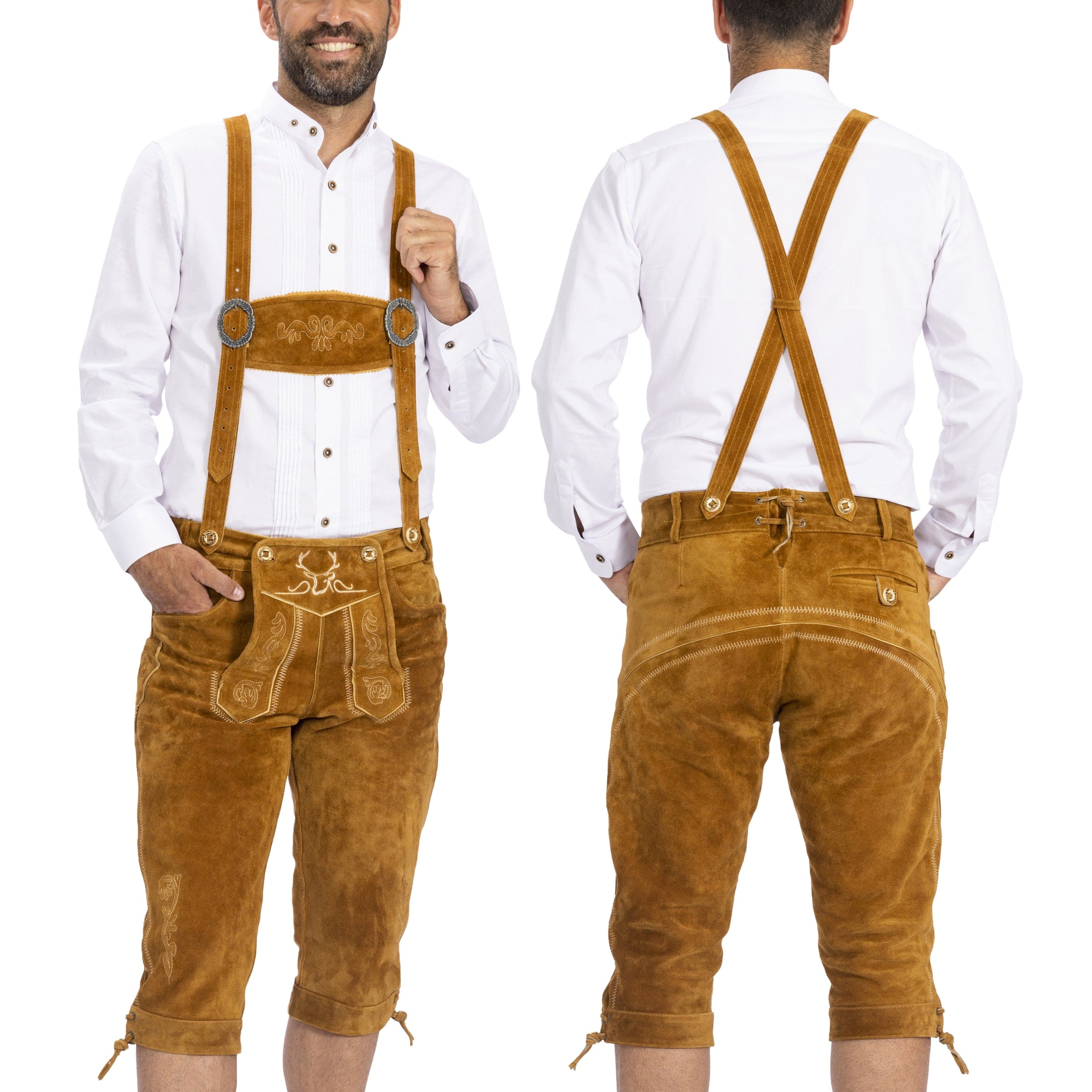This image features a man modeling a distinctive outfit, focusing primarily on his torso down to his knees, with the face and legs partially cut off. The man's attire includes a white long-sleeve button-up shirt with a standing collar. He has a short brown beard flecked with gray. The central piece of his outfit is a pair of traditional German-style overalls made of a material that appears suede or velvety in texture. These overalls are mustard brown in color with decorative etchings, including symbols like a deer head. The overalls consist of two thin straps connected by a brown patch, secured with circular buckles on each side. The pants, detailed with fancy stitching and carvings, end just below the knee and feature a single pocket on the right side at the back. In the back view, the straps cross each other, and the pants exhibit curved stitching across the buttocks.